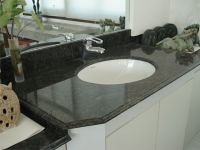A small, intimate photograph captures a home restroom's sink area. The centerpiece is a pristine white porcelain sink, seamlessly integrated into an elegant black marble countertop. Below, stark white cabinets provide contrast and storage. The sleek stainless steel faucet, complete with a single handle for temperature control, emerges from a matching black marble backsplash, exuding modern sophistication. A mirror above reflects an obscured glimpse of the rest of the room, hinting at its cozy dimensions. To the right of the sink, some towels are discernible, adding a touch of warmth, while to the left, a charming wooden owl figure perches partially visible on a white surface, offering a whimsical touch to the serene and polished environment.